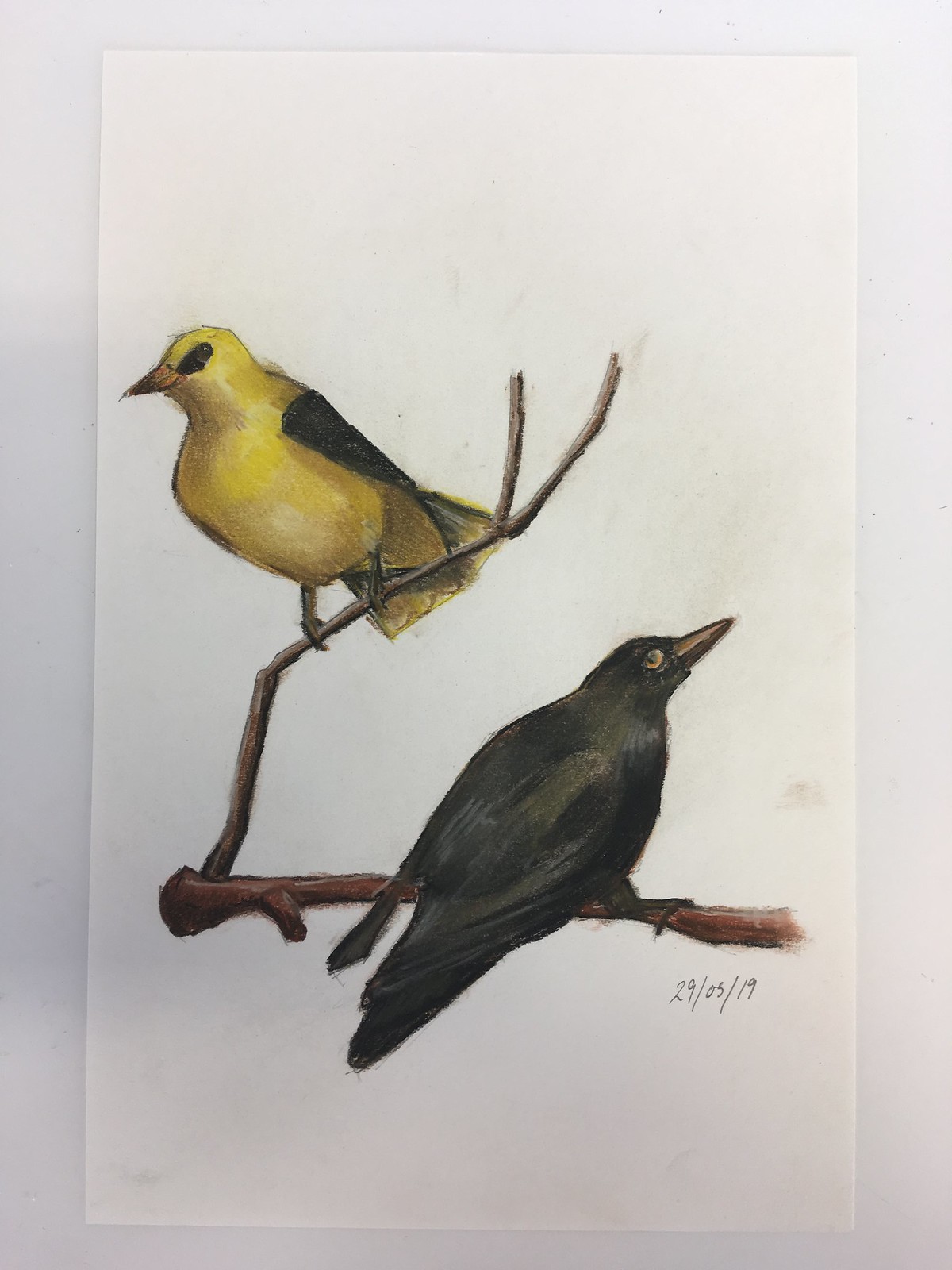A meticulously crafted drawing on sketch paper depicts two birds perched on a V-shaped branch tilted to the right. The birds are oriented oppositely, with the yellow bird on top facing left, and the black bird beneath it facing right. The open part of the V, formed by the branch, points to the right, while the branches converge on the left side of the drawing. Positioned on a white desk with a clean, white background, the detailed image includes a date inscription, "29/05/19," situated just above the black bird on the right side.